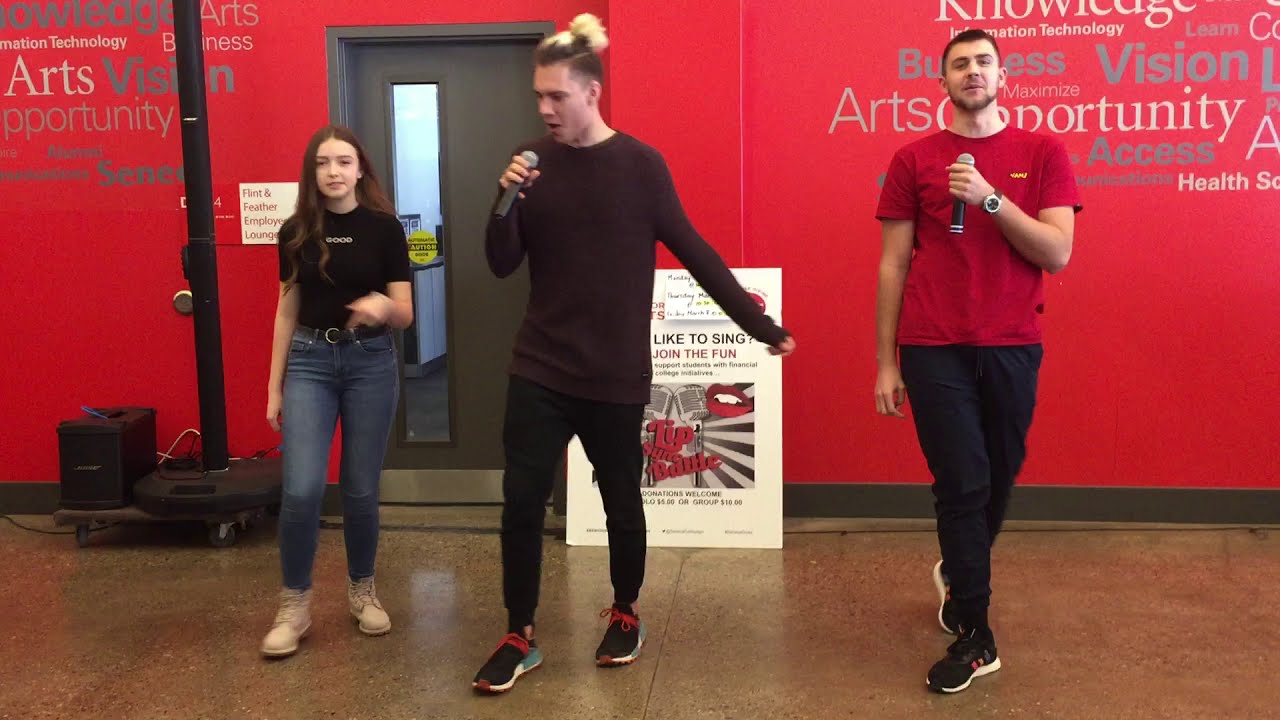In this vibrant photograph, three light-skinned individuals perform enthusiastically in an indoor art fair or auditorium-like setting. The backdrop is a striking red wall adorned with various motivational and educational words such as "art," "vision," "knowledge," "health," and "access." The text is scattered prominently across the wall, more concentrated in the top right and left corners, alongside several signs—one mentioning "Flint and Feather Employee Lounge" and another promoting a "lip-sync battle" for supporting student financial initiatives.

The three performers, all positioned centrally, are standing on a tiled floor. The young female on the left sports long dark hair, a black t-shirt, blue jeans, and white sneakers. Her blurred hands suggest dynamic movement, though she isn't holding a microphone. In the middle stands a tall male with a distinctive hairstyle, his dark hair topped with bleached highlights, tied back in a man bun. He wears a dark, long-sleeved shirt—possibly burgundy—and black jeans, with sneakers. He holds a microphone, directing his performance to the audience. To the far right is another male, characterized by his short black hair and small brown mustache. He wears a red t-shirt, black sweatpants, and sneakers, also gripping a microphone. 

The energy of the moment is palpable, caught frozen under bright lights, with a white sign on the floor behind them reading "like to sing join the fun" further emphasizing the artistic and lively spirit of the event.